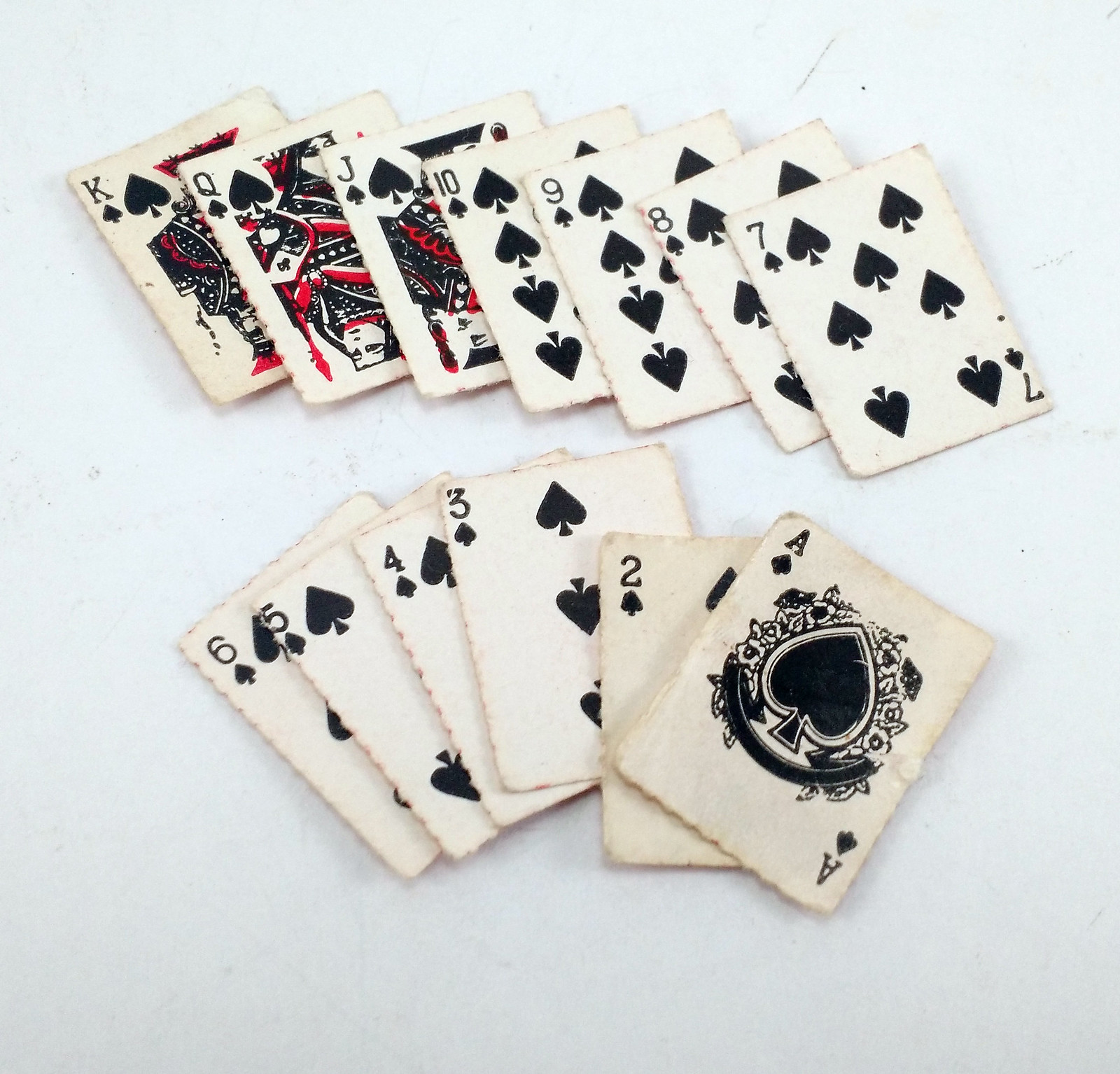A highly artistic color photograph, likely enhanced using Photoshop or a similar illustration program, showcases a visually striking arrangement of playing cards on a textured table. The cards, exclusively from the suit of spades, are divided into two distinct piles, each meticulously positioned to create an engaging composition.

In the top-left quadrant of the image, a fan-shaped array of cards leans gracefully to the left. This top pile features the King, Queen, Jack, 10, 9, 8, and 7 of spades, each card's edge partially overlapping the next and slightly obscuring the text on the cards. The face cards—King, Queen, Jack—stand out with their intricate black, white, and red illustrations.

Beneath this, another fan-shaped arrangement forms a slightly messier arc, spanning upward and downward. This lower pile includes the 6, 5, 4, 3, 2, and Ace of spades. Notably, the Ace card commands attention with its large central spade, underneath which lies a black arc and a floral design emerging from behind it.

The cards' edges are uniquely serrated, contributing to the overall dynamic and textured appearance of the photograph. Subtle pencil-like markings or possible printing flaws are visible at the top of the image, adding an element of imperfection and authenticity to the composition.